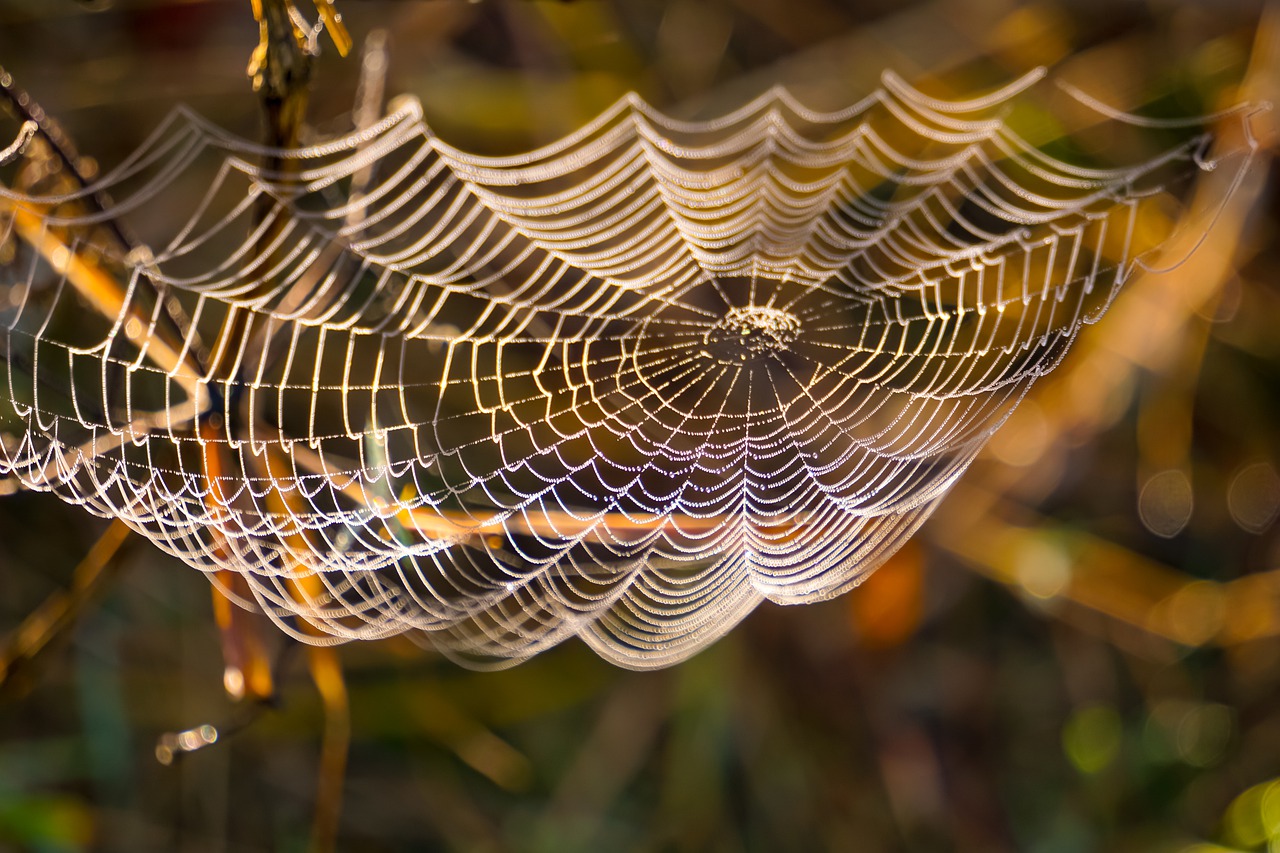This close-up photograph captures the intricate beauty of a spider's web, which spans prominently from the left to the right side of the image, occupying the upper half down to the center. The web is a vivid, bright white and designed in a concentric circle pattern, radiating outward with delicate lines and crisscrosses that catch the light, making it glisten like tiny crystals. The background, though out of focus, hints at a mix of greens, yellows, reds, and oranges, likely from vegetation such as leaves or grass, adding a warm, blurred backdrop that accentuates the clarity of the spider's web. There is no visible spider, and the web itself seems to glow with the dewy light of either the early morning or late evening sun. Near the left side, an indistinct stem can be seen, suggesting the web's attachment point, but overall, the spider's web remains the striking focal point of this serene nature photograph.